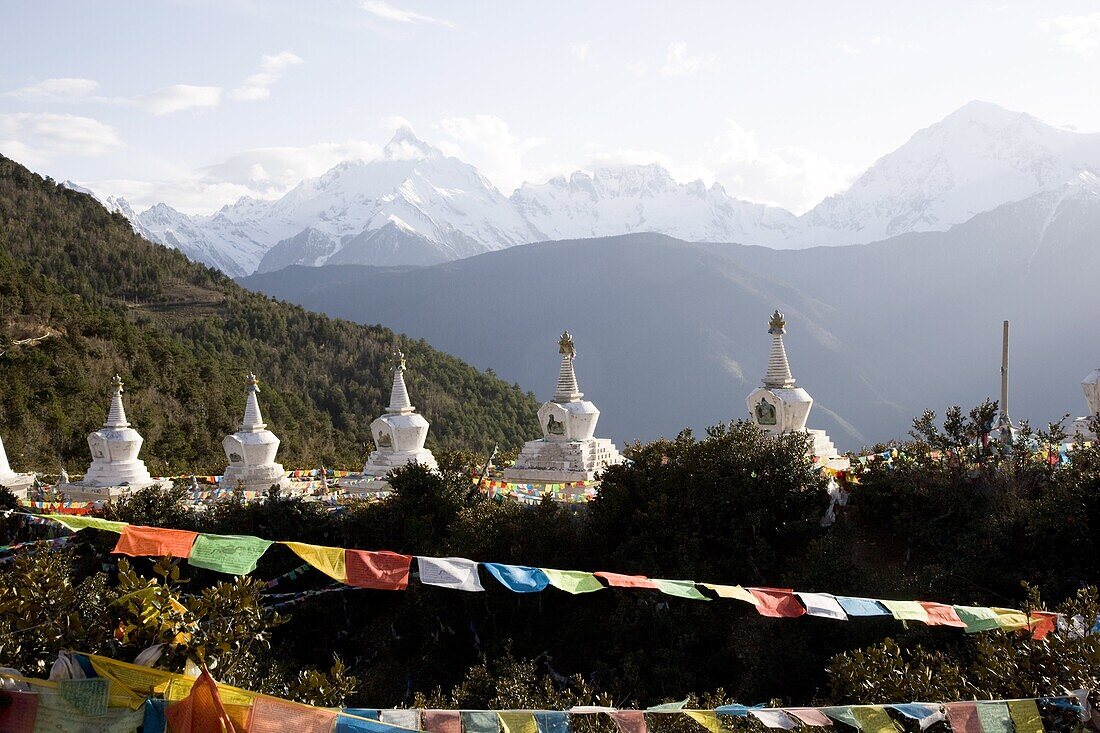This captivating image showcases a stunning mountainous landscape with a multi-layered depth. The background features a range of towering, jagged mountains covered in pristine snow, likely part of the majestic Himalayan range. In front of these imposing peaks lies a smaller, green mountain range, devoid of snow and resembling rolling hills.

Dominating the midground are five identical, white structures that resemble Tibetan monk temples or stupas. Each of these temples has a unique architectural design consisting of a large, round base that transitions into a square midsection, culminating in a triangular conical tip adorned with an emblem. These temples stand elevated on a series of steps, lending them an even more imposing presence.

In the foreground, vibrant strings of colorful prayer flags weave back and forth across the hillside, creating a striking contrast against the white of the structures and the green of the mountainside. The composition of the photo, taken from a high vantage point, offers a sweeping and detailed view of the landscape, including a road that curves around the side of the green hills. This image beautifully encapsulates the serene yet awe-inspiring beauty of a remote mountainous region, marked by cultural and natural landmarks.